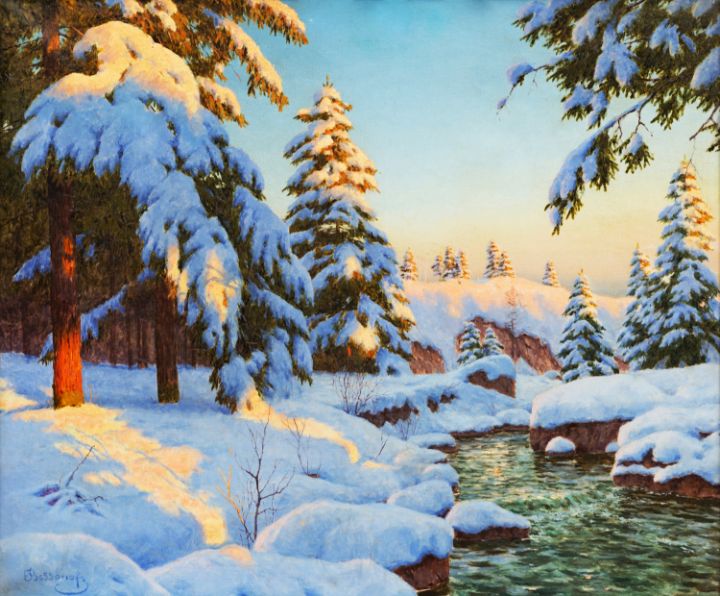The image is a highly detailed and realistic painting of a snowy forest landscape during what appears to be sunrise or sunset. The scene is dominated by numerous pine trees, all heavily laden with snow, creating a serene winter wonderland. The left side of the image features a thick tree line with coniferous trees, some of which are so snow-covered they resemble classic Christmas trees. Interspersed among the pines are small twigs and plants struggling to poke through the thick blanket of snow. To the far right, there is a small, unfrozen stream or river cutting through the forest. The green water bubbles and flows, with some rocks partially visible beneath their snow cover. The sky above is a semi-blue with a bright sun casting a golden hue on the snowy landscape, further enhancing the tranquil and picturesque scene.